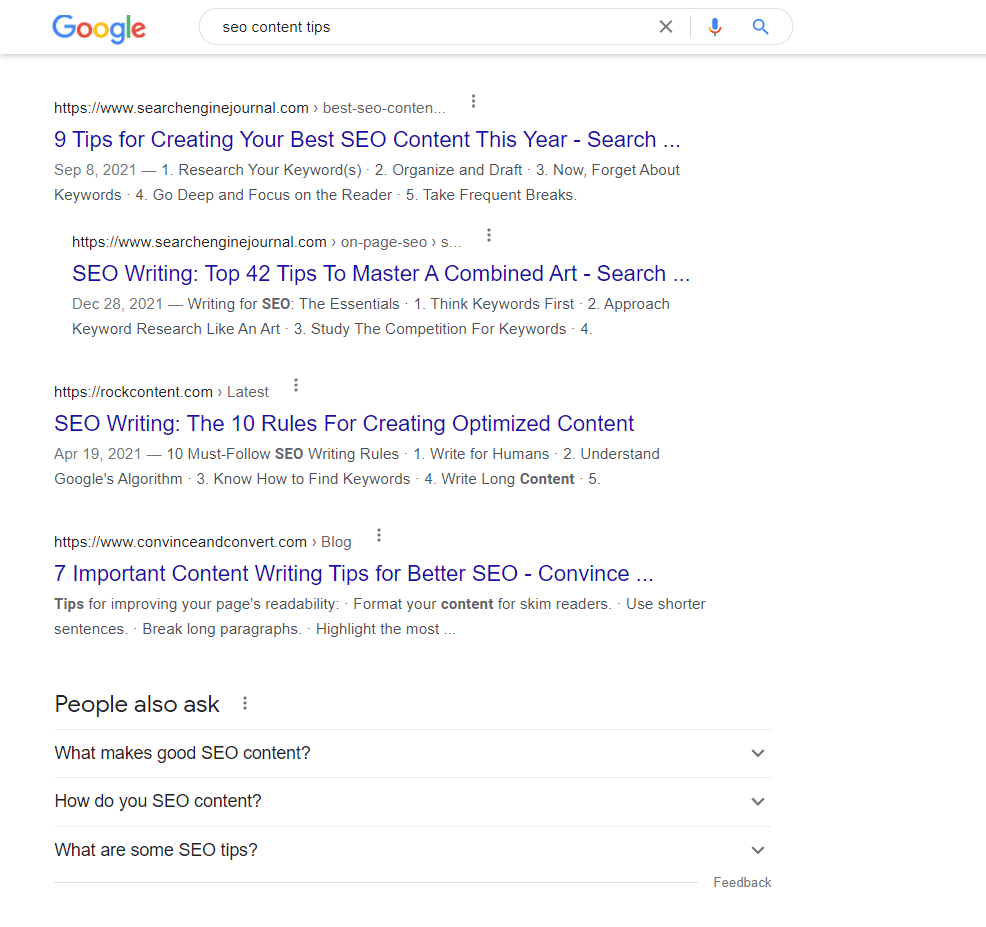The screenshot captures a Google search results page against a white background. In the upper left corner, the iconic Google logo is prominently displayed. Positioned next to the logo is the search field where the query "SEO content tips" has been entered. At the far right end of the search field, there are three icons: an 'X' for clearing the search query, a microphone for voice search, and a magnifying glass representing the search function.

Below the search field, the first search result is from https://www.searchenginejournal.com and is highlighted with blue font, stating "Here are 9 tips for creating your best SEO content this year." There is a forward arrow icon next to the snippet, indicating further information or a link to more content on the topic. Directly beneath this entry, another search result from the same website is listed. The layout is clean and organized, reflecting Google's standard design for easy navigation and readability.